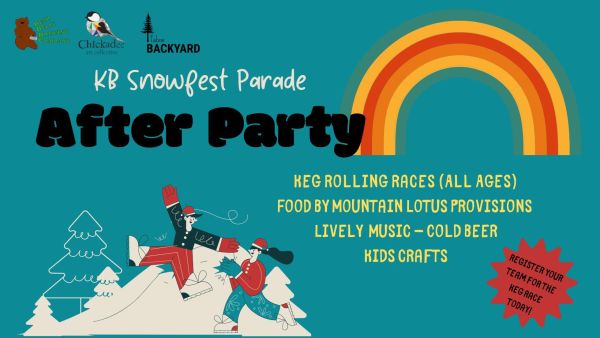This is a highly stylized cartoon poster advertising the KB Snowfest Parade After-Party. It features a prominent announcement at the top with "KB Snowfest Parade" in white text and "After Party" in black text. The background is a unique shade of turquoise blue, accented by a rainbow in the upper right corner composed of stripes in yellow, brown, orange, and yellow again—a distinct detail repeated in each description.

At the bottom left, there's an animated scene of a man and woman joyfully frolicking on a snow-covered hill. Both are dressed in winter clothing, including Santa hats with red tops and white pom-poms. The man sports a black jacket, red gloves, red pants, and white boots. The woman complements him with blue gloves, a red jacket, blue pants adorned with flower patterns, and white boots. An evergreen tree silhouette stands to the left of them.

The poster details various activities and attractions, including "Keg Rolling Races All Ages," "Food by Mountain Lotus Provisions," "Lively Music," "Cold Beer," and "Kids Crafts," reflecting a family-friendly yet lively atmosphere. A call to action in a small red star on the lower right urges participants to "Register your team for the keg race today." Additional promotional information appears in the upper left corner, including "Chickadee" and a reference to something's "Backyard," though specific details are partly obscured.

Overall, the lively imagery and inviting descriptions highlight an event packed with diverse entertainment and fun for all ages.